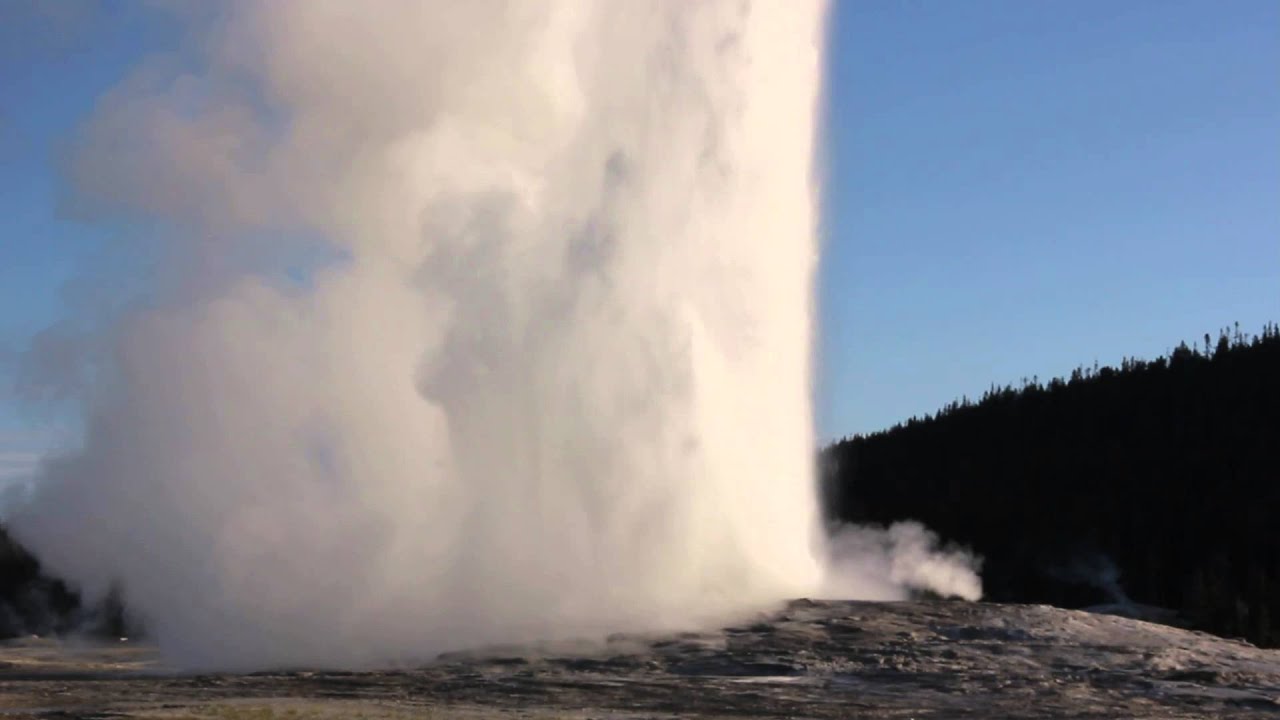This color photograph captures the iconic eruption of the Old Faithful Geyser in Yellowstone National Park against a clear, medium blue sky without any clouds. The photograph, taken in a landscape orientation, showcases the geyser near the center, emerging from a rocky, gravelly terrain devoid of plants or greenery. The powerful stream of water and steam shoots approximately 20-30 feet into the air, with the steam appearing white on the right and blending into gray on the left, forming billowing clouds. To the right, a dense forest with a variety of vegetation covers the slopes of distant hills, adding a dark green contrast to the rocky foreground. The overall style is photographic representational realism, emphasizing both the geological spectacle and the serene natural setting.